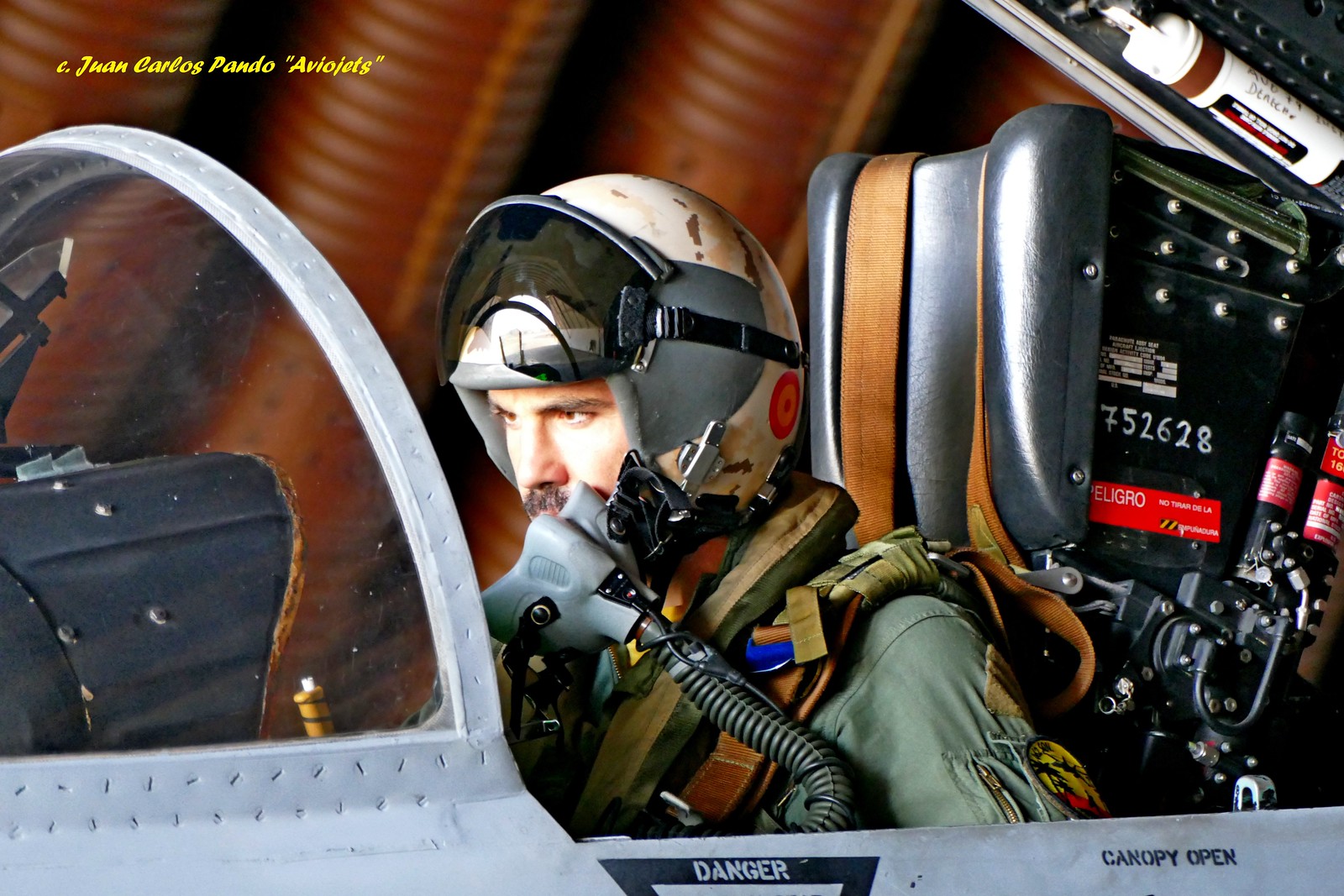The image captures a detailed scene inside the cockpit of a fighter jet featuring a pilot in full gear. The man, possibly Hispanic and with dark eyebrows, a black mustache, and dark eyes, is wearing a green-colored army uniform and a white helmet. The helmet is adorned with a large visor, which is pulled up and secured at the top, revealing his face. He is also equipped with an oxygen mask, detailed with tubes running down. 

The cockpit setting is meticulously portrayed, with the pilot seated against a silver-looking chair bristling with buttons, screws, and various control elements. Behind him, a black headrest and other equipment with a couple of wires are visible, along with a white and brown tube in the upper right corner. The pilot is intently focused on an interface element in front of him.

In the broader context of the image, the canopy of the jet is open, offering a clear view of both the pilot and his surroundings. The jet extends from the bottom left to the right of the frame, with visible markings that read "DANGER" and "CANOPY OPEN." The top left corner of the image features the text, "C. Juan Carlos Pando, AVO jets" in yellow script.